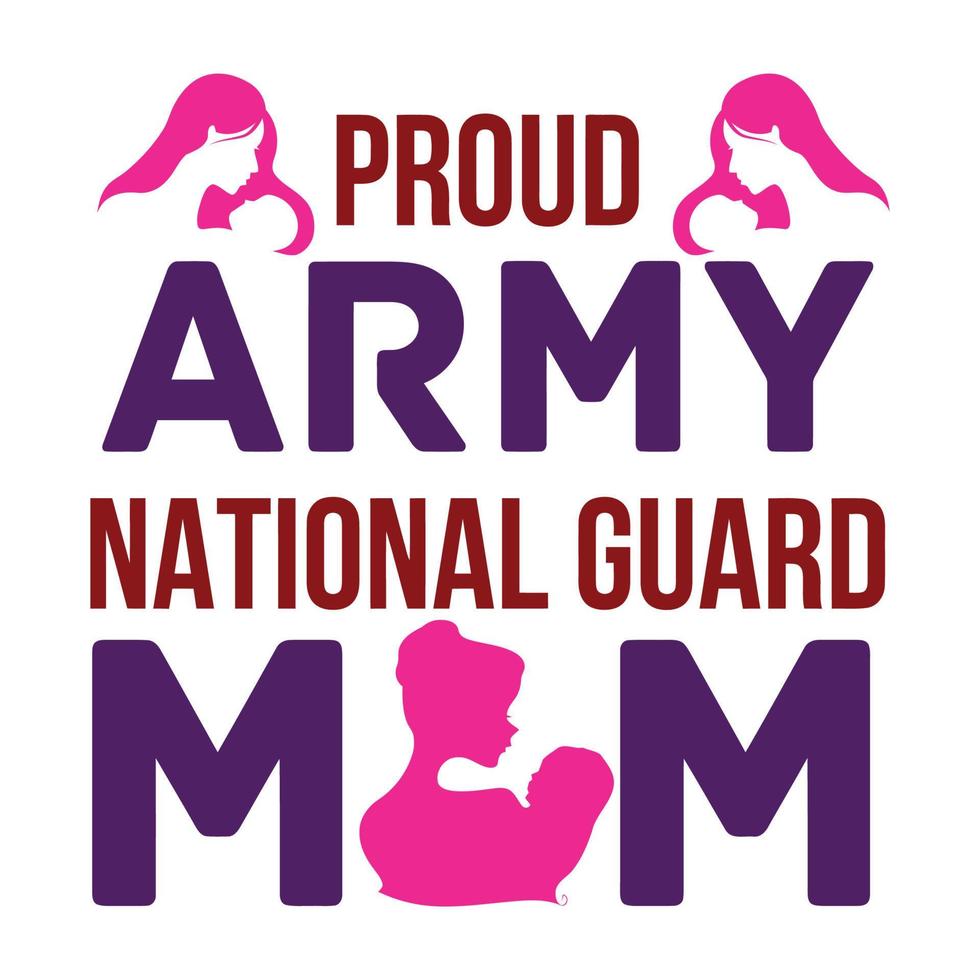This is a detailed static poster often seen on social media platforms like Facebook or Pinterest. The poster is set against a white background and prominently displays the text "Proud Army National Guard Mom" in capital letters. At the top corners, both the upper left and upper right, there's a stylized image of a woman's head leaning in to kiss a young child. These images are filled in with pink, and they mirror each other, with the mother's face on the left pointing to the right and vice versa. 

The word "Proud" sits at the top in a burgundy color, centered between the two pink images. Beneath it, "Army" is written in a large, capitalized purple font. Below "Army," "National Guard" is displayed in the same burgundy color as "Proud." The word "Mom" is at the bottom, with the two "M"s in large, capitalized purple letters. The "O" in "Mom" is substituted with another pink silhouette of a woman with her hair in a bun, cradling a child, creating a unified theme of maternal affection throughout the poster.